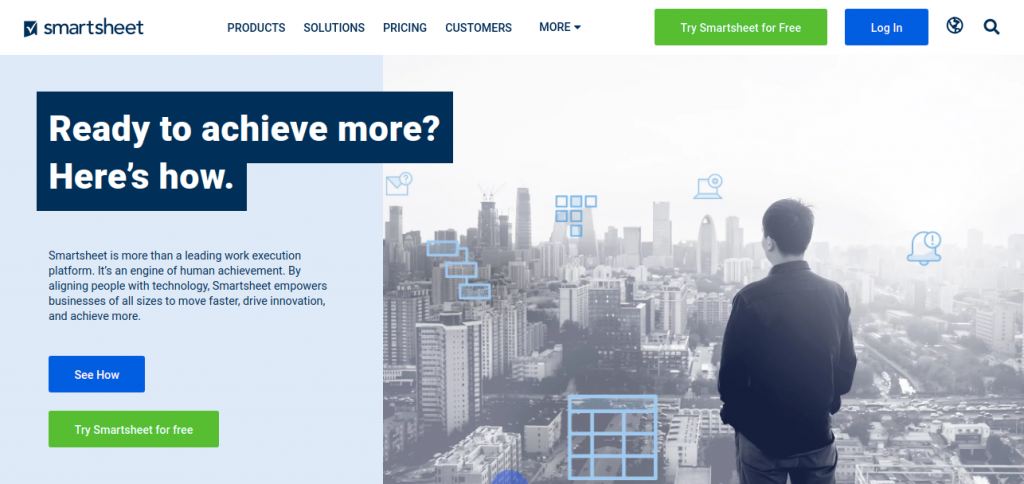The image features a user interface for Smartsheet, starting with the top left corner where there's a square with a dark blue background and a white checkmark in the center. This square is slightly indented at the bottom right. Adjacent to the square, the name "smartsheet" is depicted in lowercase, digitized dark blue font without any spaces.

To the right of the logo, a horizontal navigation menu appears, with each option in smaller, capitalized, dark blue lettering. The menu items include: PRODUCTS, SOLUTIONS, PRICING, CUSTOMERS, and MORE, the latter accompanied by a downward-pointing arrowhead indicating a dropdown list. 

On the far right of the menu bar are two rectangular icons. The first has a green background and reads "Try Smartsheet for free" in white text. The second, smaller icon, is blue and says "Log In" in white text. Next to these are two more icons: a dark gray globe and a gray magnifying glass, indicating language settings and a search function respectively.

Directly below this header, the main banner spans the width of the interface. On the left side, there's a rectangular area with a pale blue background. Within this, a dark blue label-style banner contains white text asking, "Ready to achieve more?" followed by "Here's how." in white font. Beneath the label, a detailed description in dark blue font reads: "Smartsheet is more than a leading work execution platform. It’s an engine of human achievement. By aligning people with technology, Smartsheet empowers businesses of all sizes to move faster, drive innovation, and achieve more."

Below this description, two call-to-action buttons are present. The first is a blue rectangular button with white text that says "See how." Below it, there’s a larger green rectangular button, also with white text, stating "Try Smartsheet for free."